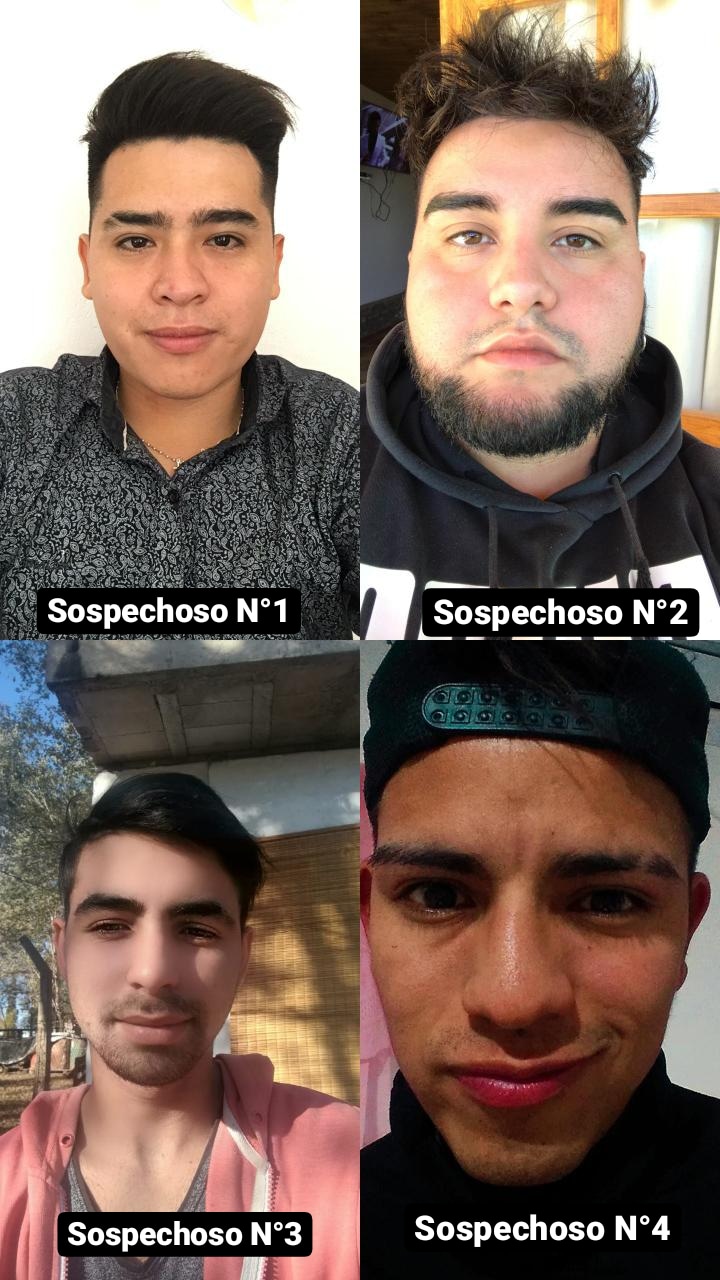This is a detailed photograph collage consisting of four portrait panels, arranged in a two-by-two grid, featuring close-up shots of men's faces. Each man is labeled with the word "sospechoso," meaning "suspect" in Spanish, followed by a number from one to four. The labels are set against a black background with white text. 

In the top-left portrait (Sospechoso No. 1), the man has short dark hair, longer on top, swept to the right, with a shaved line in his right eyebrow. He wears a gray jacket and stares directly into the camera. 

The top-right portrait (Sospechoso No. 2) shows a man with a fuller face, tousled wispy lighter brown hair, a short beard, and stubble mustache. He is dressed in a black hoodie with white writing and has an earring. 

Below, the bottom-left portrait (Sospechoso No. 3) features a thinner man with pale skin, dark hair, and five o'clock shadow. He is dressed in a gray V-neck t-shirt paired with a pink zip-up hooded sweatshirt. He gazes slightly off to the side.

The bottom-right portrait (Sospechoso No. 4) is a close-up shot of a man with darker skin and a backwards black cap, through which some wispy hair peeks. He has a smirk on his face and a shaved line in his left eyebrow. He wears a black turtleneck, looking directly into the camera.

Three of the portraits appear to be taken indoors, while one seems to be outdoors. The men are all likely of Latino descent, and their intense gazes and varied expressions contribute to the intriguing narrative of the collage.